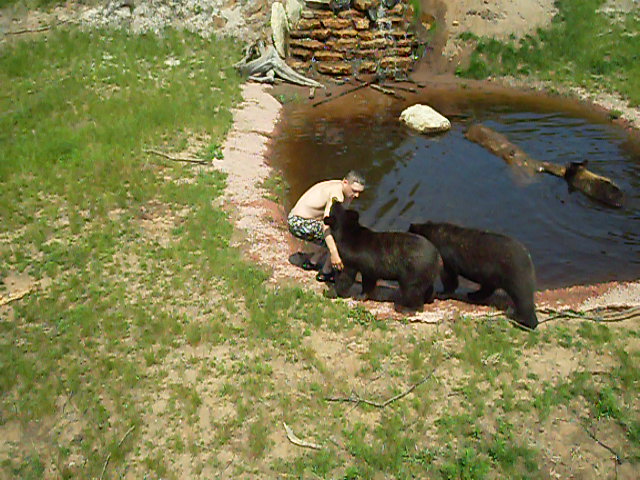In this detailed colored photograph taken outdoors, the scene centers around a small, circular, man-made pond with dark, murky water. A stone wall background features a cascading, man-made waterfall that pours into the pond. The perimeter of the pond is lined with light beige rocks, forming a low wall with steps leading up, surrounded by a sparsely grassed area with patches of bare earth. 

At the edge of the pond, two young black bears are interacting with a shirtless man in black swim trunks. The man is squatting and appears to be affectionately wrapping his arm around one of the bears' necks. The other bear is standing just behind it, both bears sniffing and engaging with the man. In the pond, there's a large white-gray rock and a floating log. Additionally, a third, smaller brown bear is seen near the log, seemingly swimming. The man’s familiarity with the bears suggests a friendly and safe interaction. The image beautifully captures a unique moment between humans and wildlife in a controlled, naturalistic setting.